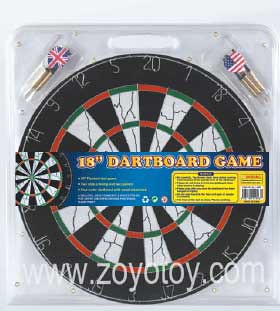The image depicts a brand new dartboard in its original packaging, enclosed in a clear plastic clamshell container. The circular dartboard features a black background patterned with alternating black and white wedges that have a distinct crackle design. Concentric circles guide the eye toward the bullseye at the center. Numbers from 1 to 20 are arranged around the exterior of the dartboard. Attached to the packaging is a blue label that reads "18-inch Dartboard Game." Two sets of darts are included in the package; one set with flanges adorned with the American flag and the other with the Union Jack flag of the UK. The clear plastic packaging has a convenient hook for hanging it on a store rack. A watermark that reads www.zoyotoy.com stretches across the bottom of the photograph.